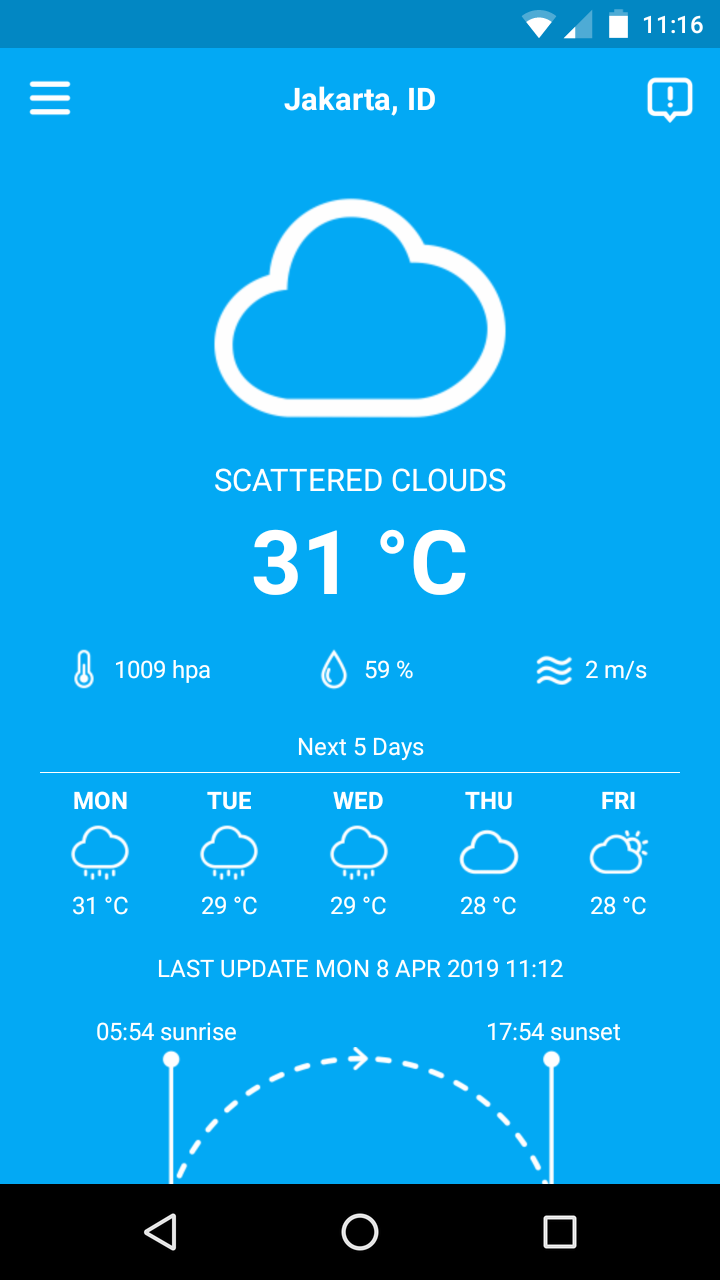This screenshot displays a weather page for Jakarta, Indonesia, featuring detailed weather information in an organized layout. 

At the very top, typical phone status icons are visible, including Wi-Fi, signal strength, battery percentage, and the current time. Just below, on a light blue background, the weather conditions for Jakarta are presented. The title "Jakarta, ID" appears in small white font.

Centrally placed is a large, simplistic clipart of a cloud, outlined in white. Directly below, the text "SCATTERED CLOUDS" is displayed in all capital letters. The current temperature is prominently shown as "31°C" in large white numbers. Right underneath the temperature reading, there is a thermometer icon followed by "1009 HPA," indicating the atmospheric pressure.

Further details include a water droplet icon with "59%" next to it, representing humidity levels. To the far right, an icon of waves is accompanied by "2 m/s," denoting wind speed. 

Below these main details, there is a forecast for the next five days, depicted in a horizontal line. For Monday, a rain cloud icon is shown with a temperature of "31°C", while Thursday, lacking any rain icon, shows "28°C".

The bottom section provides additional information: the last update was on Monday, April 8th, 2019 at 11:12 AM. Additionally, there are sunrise and sunset times, visually separated by a semicircular dashed line in the middle.